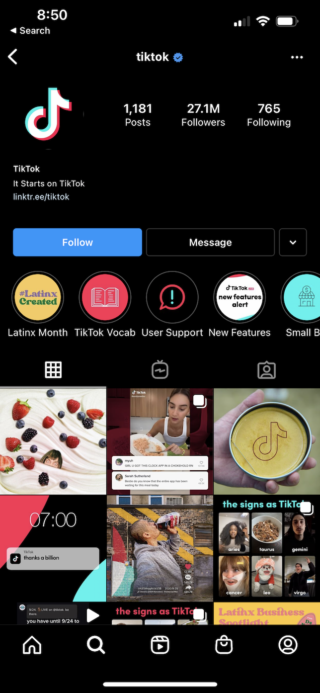The image is a placeholder icon indicating a failed image load. It features a small, folded corner of a page with a sky and cloud in the background. A diagonal line crosses through it, signifying a broken link or missing file. The remaining space, where an image should have been displayed, is entirely white. This placeholder appears frequently on the internet when an image fails to load due to various reasons such as the file not existing or server issues.